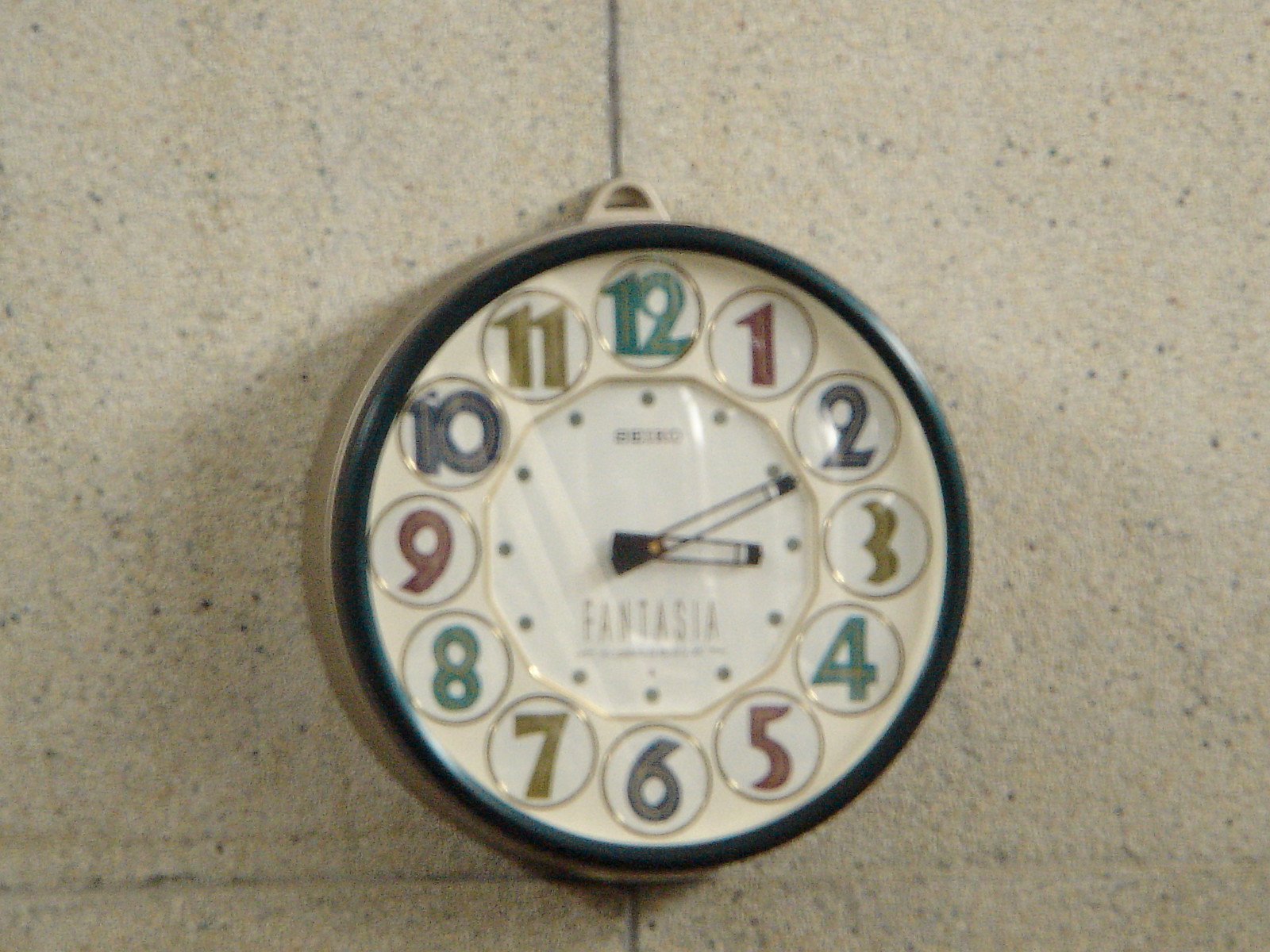This image features a close-up of a small, circular clock mounted on a white, sandy-textured wall, which possesses subtle black speckles and a distinct black line running vertically down the center. The clock hangs directly on this black line from a tab or hook at its top. The clock itself has a layered appearance starting with an outer blue beveled border, followed by a slightly inset yellowish-white border, and finally, a pure white face that hosts the clock's display features. The clock's numbers are vividly multicolored, arranged in a pattern of green, red, blue, and gold, and run in a clockwise direction. Each number is accompanied by small dots arranged in a smaller circular path inside the clock's main face. The clock's hands are wire-framed and black, with the minute hand being notably long and slender, while the hour hand is shorter and stouter. Below the hands, the text "MANTASIA" is visible. The entire image has a slightly blurry and out-of-focus quality. The time displayed is approximately 3:10 or 3:11.